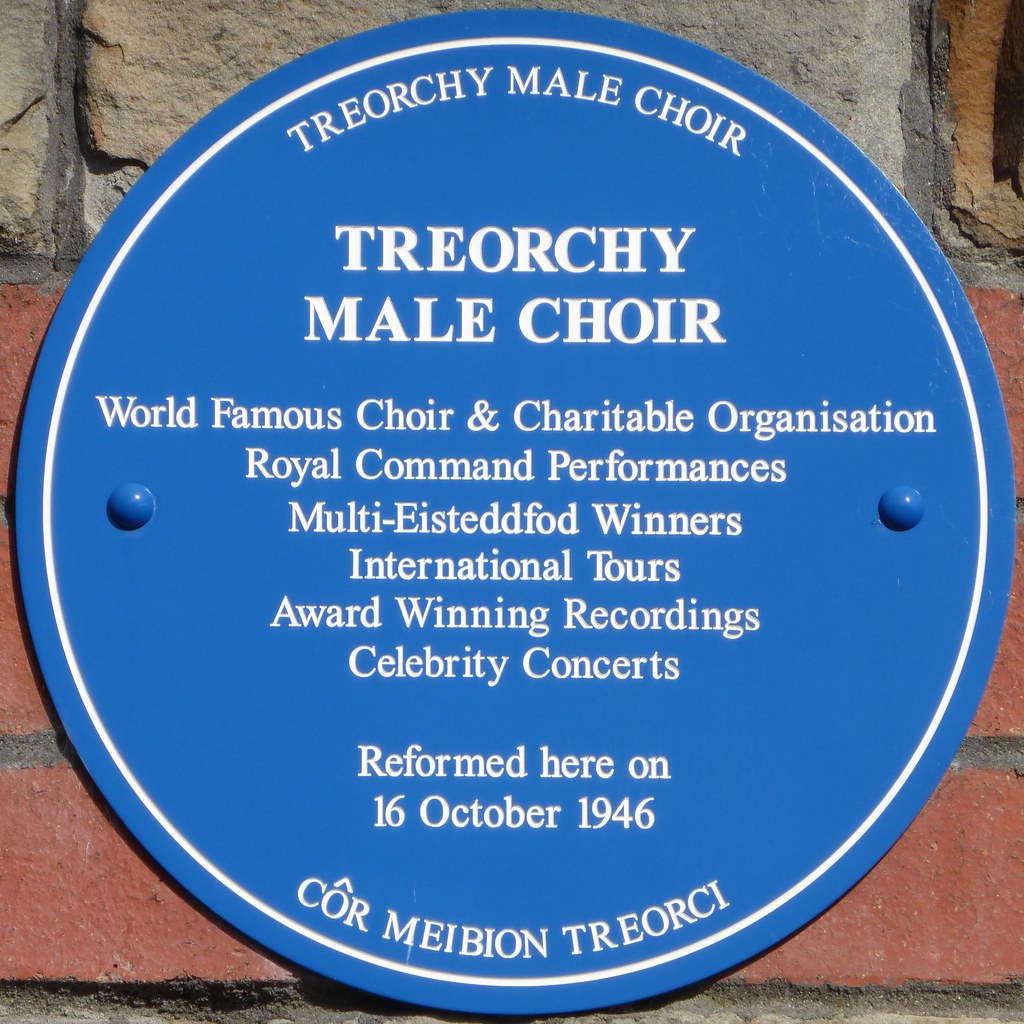This full-color photograph features a circular blue plaque firmly attached to a brick wall. The plaque, which provides detailed information, has a thin white border and contains predominantly white serif text. The text is organized in a clear, readable format, likely in bold Times New Roman, and reads:

"Treorchy Male Choir, Treorchy Male Choir, World Famous Choir and Charitable Organization, Royal Command Performances, Multieisteddfod Winners, International Tours, Award-winning Recordings, Celebrity Concerts. Reformed here on 16th October 1946."

Beneath the English text, there is a statement in Welsh, spelled out as "Côr Meibion Treorchy." The plaque commemorates the renowned choir's rich history and various accomplishments, emphasizing its global tours, award-winning recordings, significant performances, and charitable status.